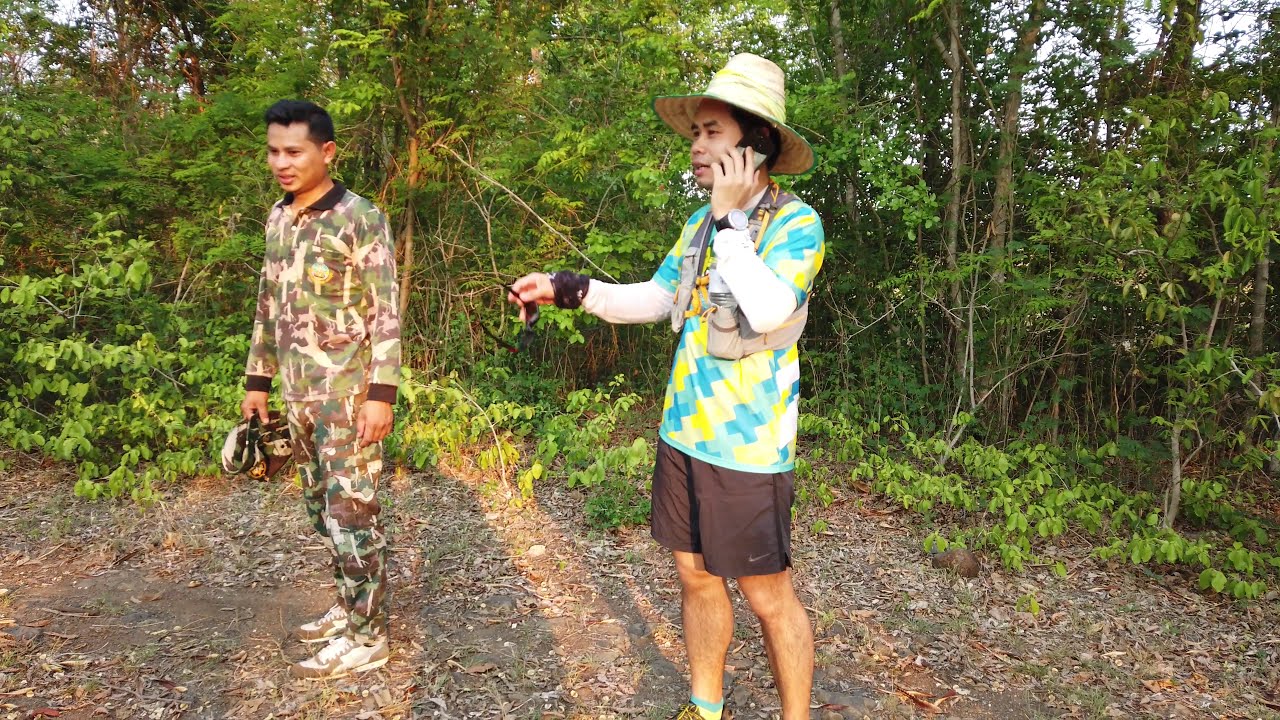The image portrays two Asian men standing outdoors on a dirt and leaf-covered ground in front of a dense clump of bright, tropical-looking trees, suggesting a rural area, possibly in Thailand. The first man, who captures initial attention, is attired in black Nike shorts and a distinctive, brightly colored short-sleeved shirt adorned with alternating blue and yellow X patterns, over a long-sleeved white shirt. He accessorizes with a large face watch on his right hand, a phone held to his ear with his left hand, sunglasses, and a small backpack with a water bottle. His head is protected by a wide-brimmed straw hat featuring a green brim and a yellow ribbon. The second man, positioned to the left, is clad in green and brown camouflage attire with a collared long-sleeved shirt and matching pants, with brown cuffs on the sleeves and neckline. He holds a camo-covered hat and wears gray and white athletic shoes. He appears to be smiling subtly while glancing downward. The vibrant foliage and traditional elements in their attire accentuate the photo's likely setting in rural Thailand.